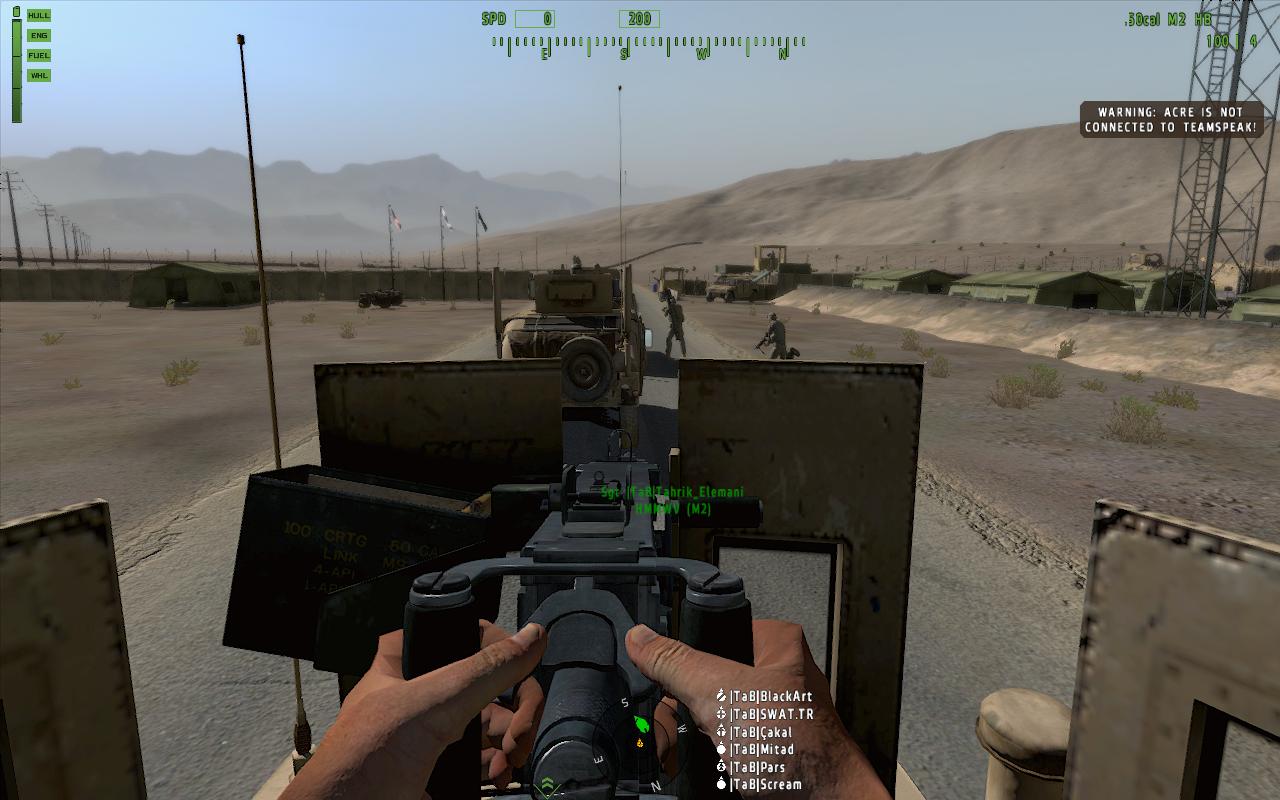In this image, we see a dynamic scene from a first-person shooter video game with a military theme. At the center, the main character is manning a mounted machine gun turret, likely attached to some form of armored vehicle that resembles a tank. The character has both hands securely placed on the gun turret, aiming straight ahead as if preparing for engagement. The surrounding environment is a vast, sandy, and barren landscape, accentuating the desolate setting of the game. Ahead in the distance, various other vehicles are visible, suggesting a convoy or battalion on the move. On the right side of the image, several green military tents are set up, indicating a makeshift base or camp. The overall scene conveys a sense of preparation for an imminent conflict as the character's vehicle begins its journey down a sandy path.